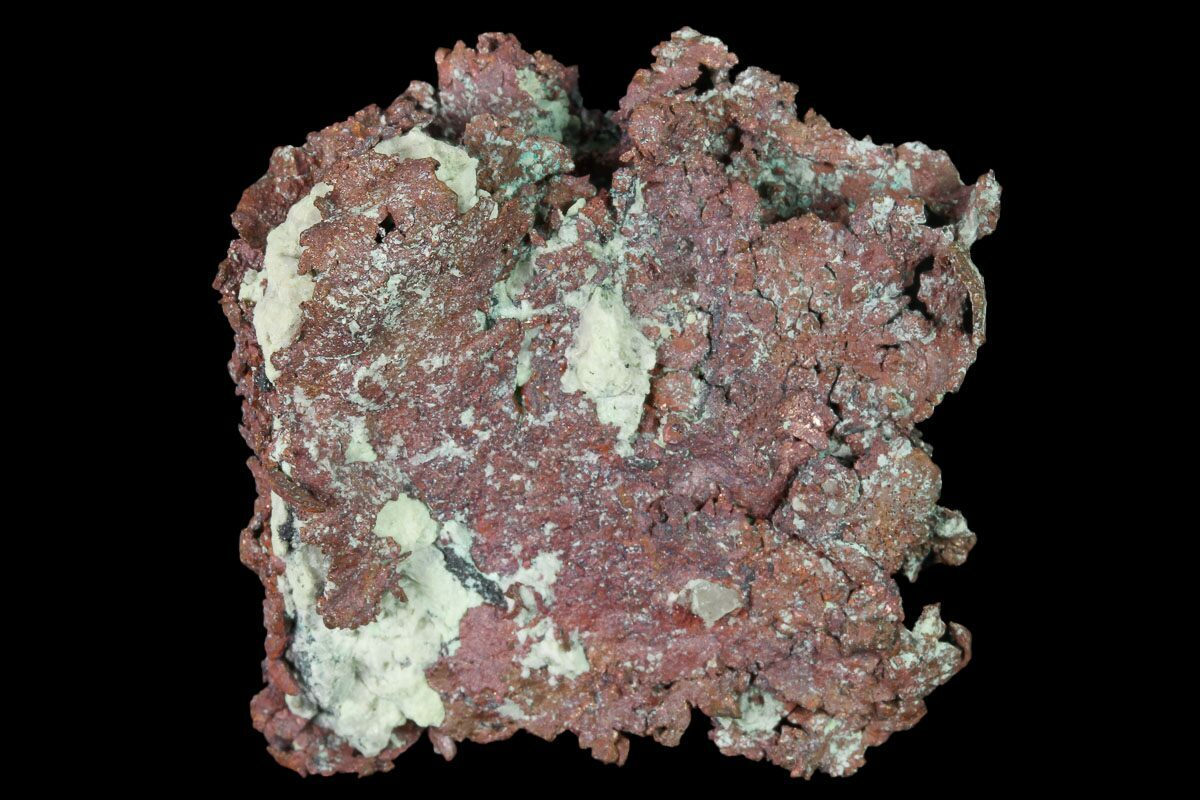The image displays a close-up of a presumably natural element against a pitch-black background. The focal point of the image is a large, irregularly shaped stone or mineral that evokes the texture and color of cooked ground beef. The object is primarily red with a complex pattern of cracks and crevices, interspersed with patches of off-white material. Additionally, there are accents of brown and black shadows, enhancing its earthy appearance. Smaller rock fragments appear embedded within its surface, hinting at a composite structure. The object presents a vague square shape with highly irregular, uneven edges, and various nooks and holes. Well-lit and prominently displayed, it suggests a possible museum exhibit, emphasizing its ancient and hard nature.